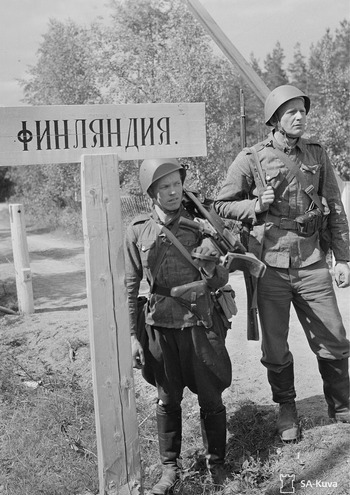This black and white photograph, likely from the World War era, depicts two Russian soldiers standing on a grassy field adjacent to a dirt road, set against a backdrop of leafy trees and dense vegetation, suggesting a rural, forested area. The soldier positioned on the far right holds a rifle resting on his right shoulder and gazes intently into the distance. Meanwhile, the soldier in the center, notably shorter and holding a gun, shares a baffled expression as if reacting to something unexpected. Both are clad in full army uniforms, including helmets and apparent backpacks, emphasizing their readiness for duty. To their left, a white wooden sign with Russian writing stands on a post, though the mirrored text is difficult to decipher. Additionally, a second white wooden pole is visible behind them. The bottom right corner of the image features a clip art depiction of a castle labeled "S.A. Kuva," adding an unexplained element to the scene.